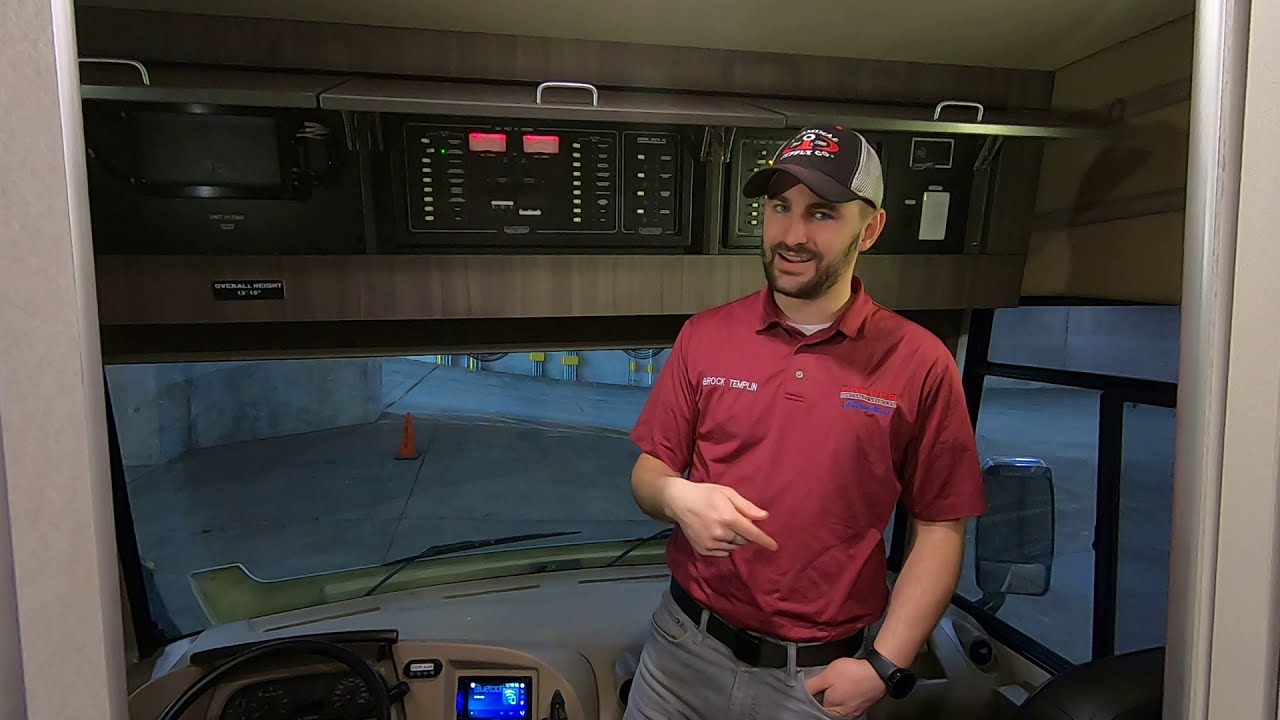The image captures the interior of a large vehicle, such as a semi-tractor trailer or an RV, predominantly featuring muted tan and gray tones. Inside the cabin, a man stands just right of center, facing the viewer with a slight smile. He appears to be in his 30s, with a brown beard and mustache, wearing light gray jeans, a black belt, and a red polo shirt. The shirt has white text on the right breast and red, white, and blue text on the left, suggesting intricate branding or logos. On his left wrist, he sports a black wristwatch. Atop his head, he dons a black and white baseball cap adorned with red and white graphics featuring small, unreadable text. Above the driver’s area, several panels are open, revealing various electronics and switches. To the right of the steering wheel in the dash is a digital screen. Through the windshield, an indoor parking garage is visible, with a prominent traffic cone centered in the view.